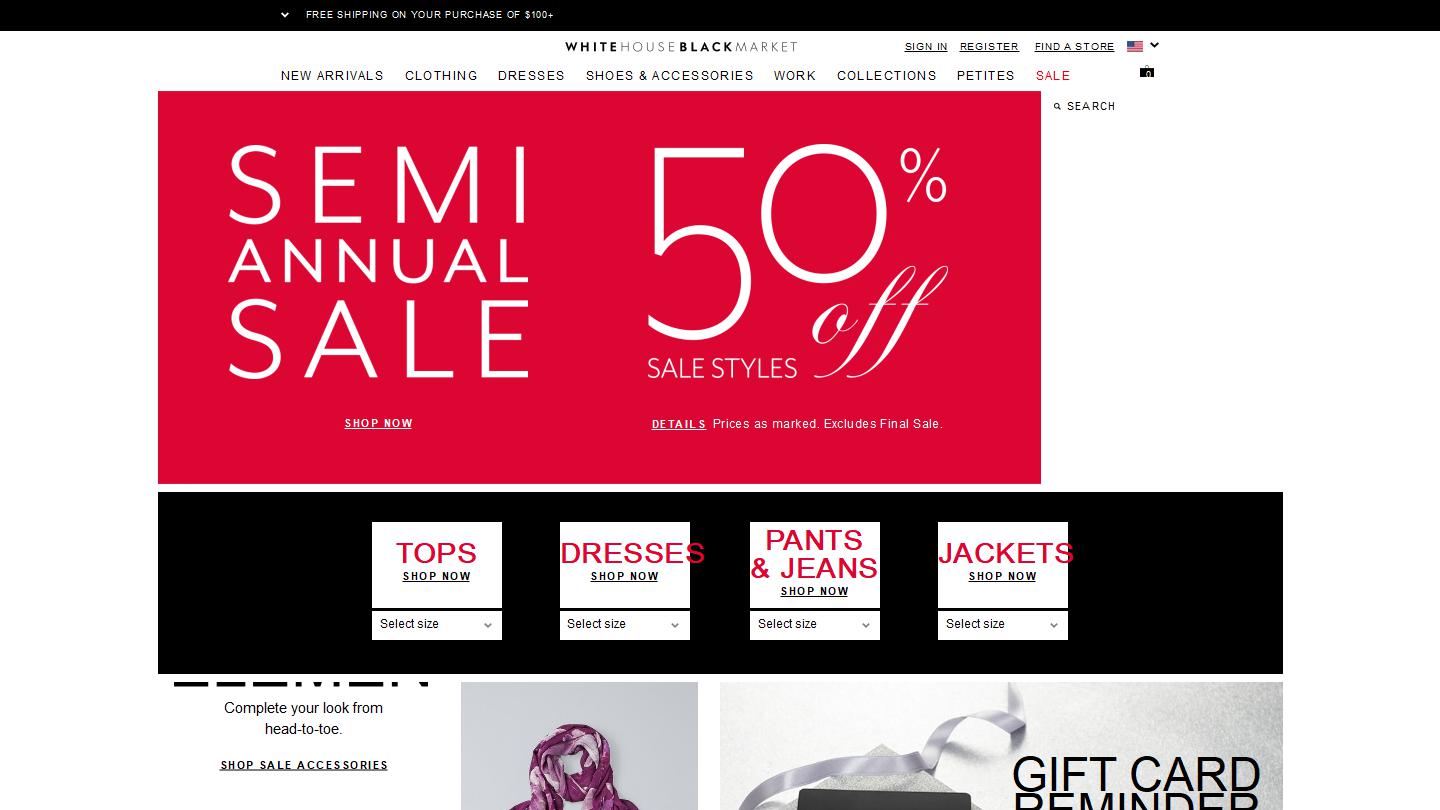This webpage belongs to the website "White House Black Market." At the top, there are options to sign in or register and a store finder. The main advertisement in the center features a prominent announcement about a "Semi-Annual Sale" with "50% Off Sale Styles." Although the layout of the ad seems a bit cluttered, the message emphasizes significant discounts. Below this advertisement, there are several clickable sections for easy navigation, including "Tops," "Dresses," "Pants and Jeans," and "Jackets." Towards the bottom of the page, there is additional advertising promoting gift cards and accessories, encouraging customers to complete their look from head to toe. Accessories likely include items such as belts and jewelry. The website can be accessed at whitehouseblackmarket.com.